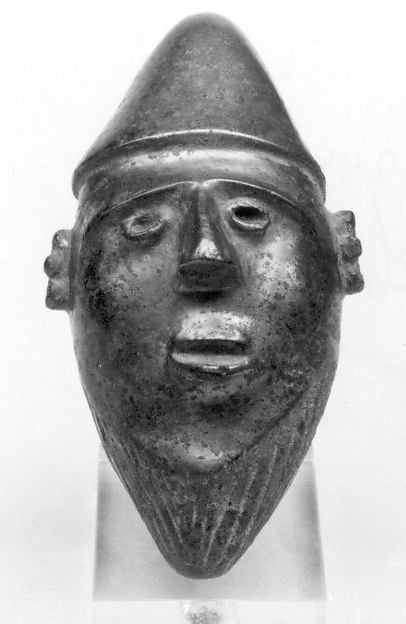This photograph showcases an intricate and ancient-looking face mask, appearing to be an artifact from antiquity. The mask, which seems to be constructed from metal, exhibits a dark silver or lead-gray tone with varying highlights and shadows causing some parts to shine. Strikingly detailed, the mask is designed with a conical mushroom-shaped head and a pointed chin, giving it a distinctive, elongated appearance. The face has hollowed-out eye sockets, a defined nose, and lips carved out with a noticeable gap between the upper and lower sections. Protruding from each side of the head are ear-like shapes that add to its realistic yet eerie presence. Set against a faint, light white background, the whole composition gives off a striking, almost haunting, visual effect, reminiscent of a piece of ancient art.